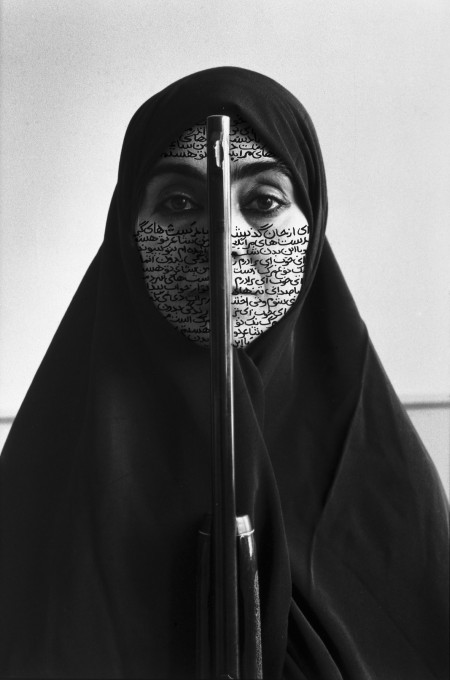This is a highly detailed and dramatic black-and-white portrait of a woman, characterized by its realistic and intense depiction. The woman is wearing a full head and body covering, a black robe resembling a burqa or hijab paired with an abaya, indicative of very conservative Muslim attire. Her face, the only visible part of her, is overlaid with Arabic text, covering everything except her strikingly large and dark eyes. The Arabic script spans her forehead, around her eyes, and down to her lips and nose. She holds a shiny black rifle vertically in front of her face, with the barrel extending from her forehead to just beyond her chin. Her expression is solemn and sad, with an intense and almost haunting gaze directed straight into the camera, suggesting a nuanced narrative of silence and protest. The background is a stark, light grey, casting the woman’s serious demeanor into sharp relief against the empty space behind her.